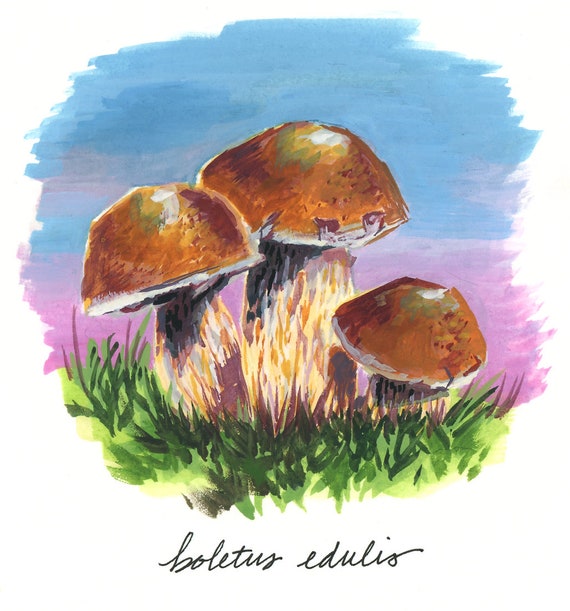The image features a detailed marker drawing on a white background, skillfully mimicking the appearance of watercolor. The top half of the scene is colored in blue, suggesting a serene, open sky, while the bottom half transitions into a light purple hue, hinting at the onset of sunset. The focal point of the artwork is a group of three wild mushrooms, specifically Boletus edulis, prominently labeled in cursive black at the bottom. These mushrooms rise from a patch of lush, dark green grass, indicating a well-cared-for environment.

The central mushroom is the tallest, boasting a brownish-orange cap and a lighter, whitish-yellow stem. To its right stands the smallest mushroom, approximately half the height of the central one. The third mushroom on the left is slightly larger than the one on the right but still smaller than the central mushroom. The mushroom caps exhibit a subtle gradient, with hints of green blending into the brown. Underneath the caps, the stalks display a whimsical array of colors, including purples and grays, adding an artistic flair. This vivid, harmonious composition offers a snapshot of nature, marrying botanical accuracy with creative expression.